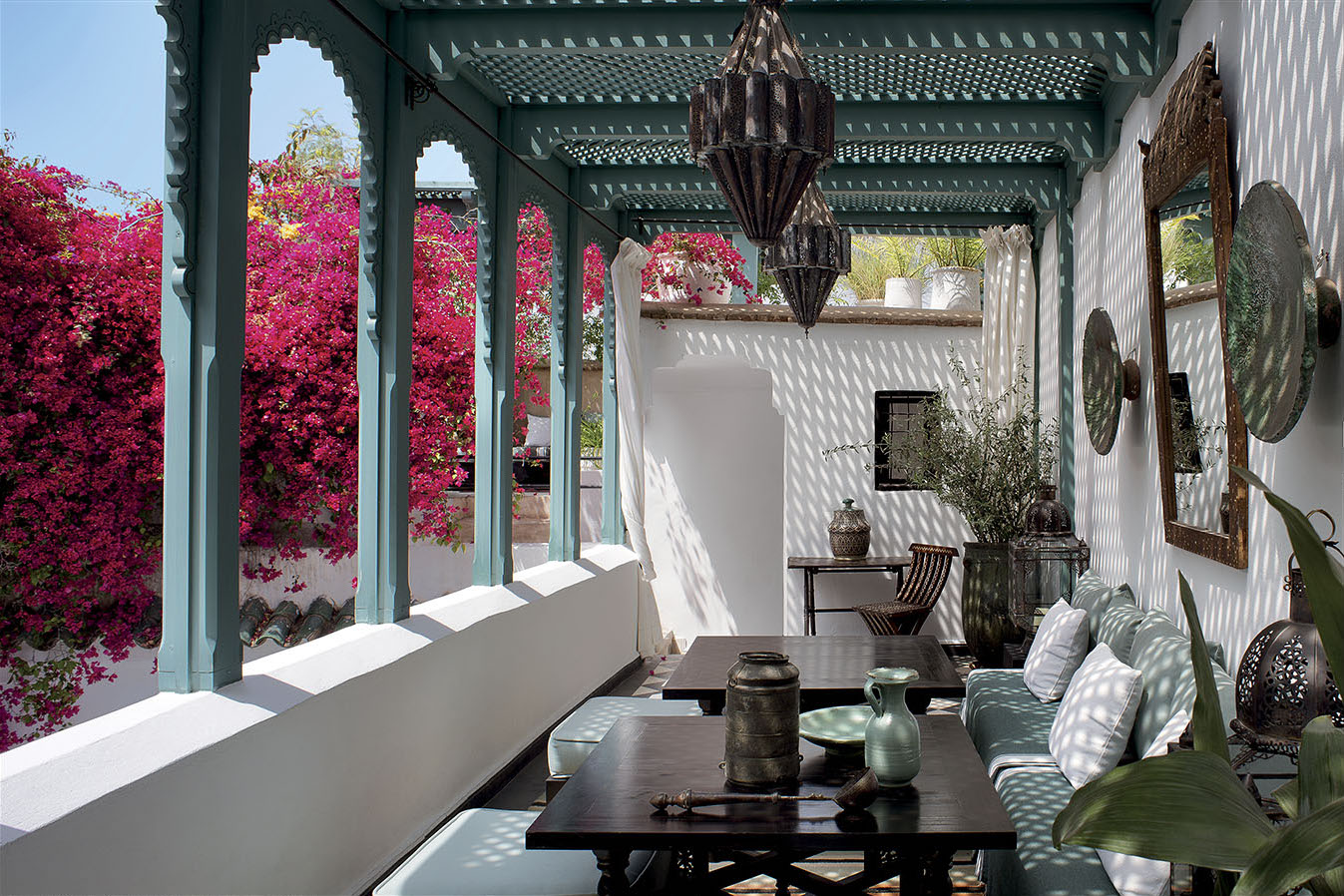The photograph captures a charming balcony scene bathed in sunlight streaming through a small grid canopy. The roof, resembling a gazebo with a patterned structure that partially masks the light, creates a serene ambiance. Blue pillars and archways frame the balcony, their hue matching the light blue couches adorned with pillows. Toward the left, the balcony overlooks a lush garden adorned with vibrant greenery, possibly with trees bearing red leaves or reddish-pink flowers.

Centered within the balcony are two brown, square tables and a smaller table at the far end, paired with a wicker seat. The tables are neatly positioned near the couches, with one of them holding a light blue metal pitcher. On the right side, near the tables, the comfortable couches invite relaxation. A mirror on the wall enhances the space, reflecting the ambient light and decor. The balcony's white walls contrast with the blue furnishings and the multitude of plants and decorative elements scattered around, adding to the aesthetic appeal. Two unique hanging lights from the ceiling provide additional charm to this picturesque, potentially restaurant-like patio setting.